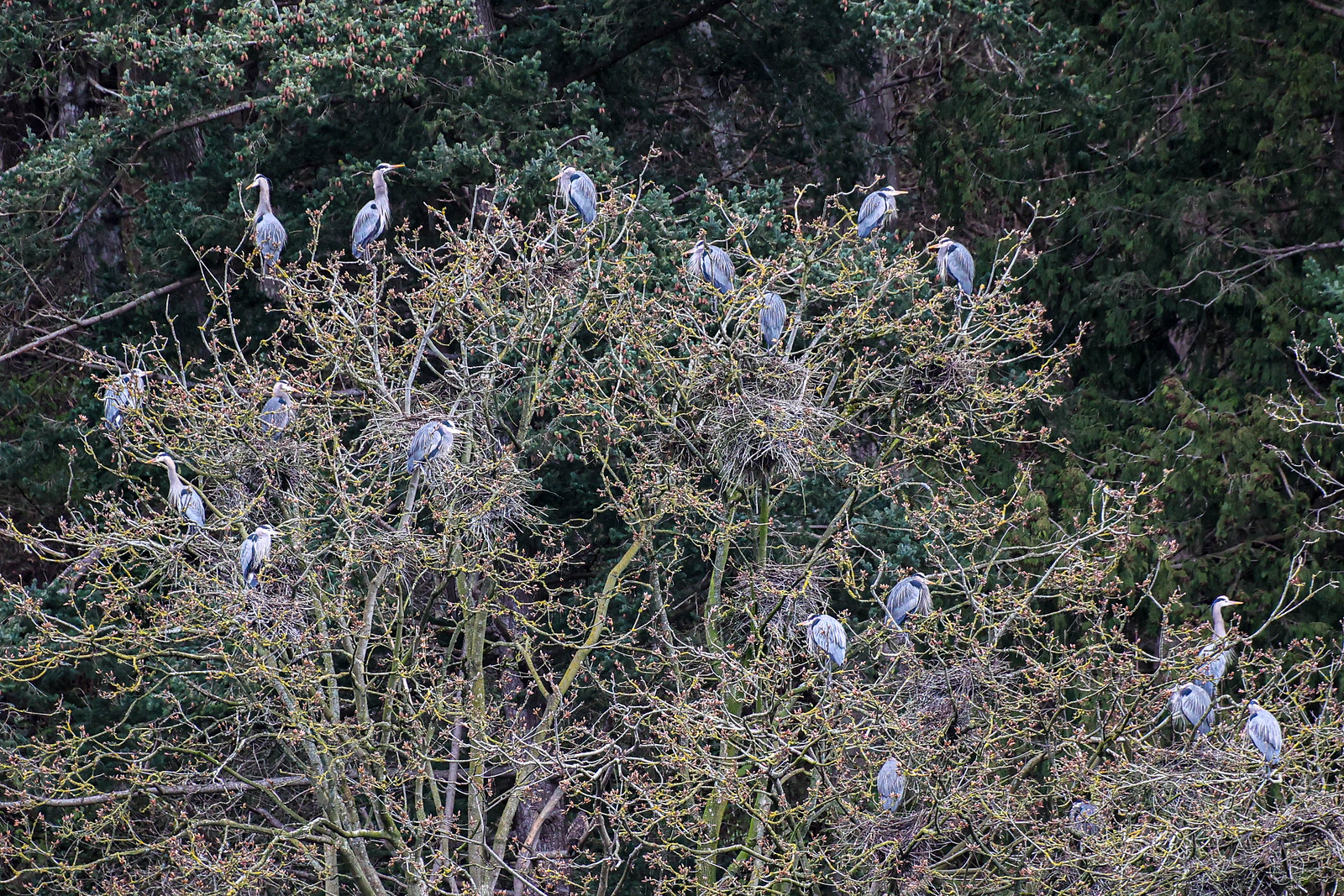This outdoor photograph captures a striking scene of numerous large birds, likely cranes or storks, perched atop the branches of a craggy, sparse tree that appears unhealthy and potentially dead. The tree itself has a skinny green trunk with yellowish branches and very few, if any, leaves, along with forlorn brown flowers. The birds, numbering around 17, boast long necks, white feathers with gray markings, orange or yellow beaks, black breast markings, and vivid sky blue wings. They face various directions, adding a dynamic element to the composition. Surrounding the sparse tree is a lush backdrop of taller trees brimming with green leaves and vibrant flowers, emphasizing the contrast between the vitality of the background and the starkness of the tree the birds inhabit. The photo, taken from a high angle possibly using an elevated position or a drone, captures both the detailed textures of the foreground tree and the encompassing verdant forest under a sunny sky.